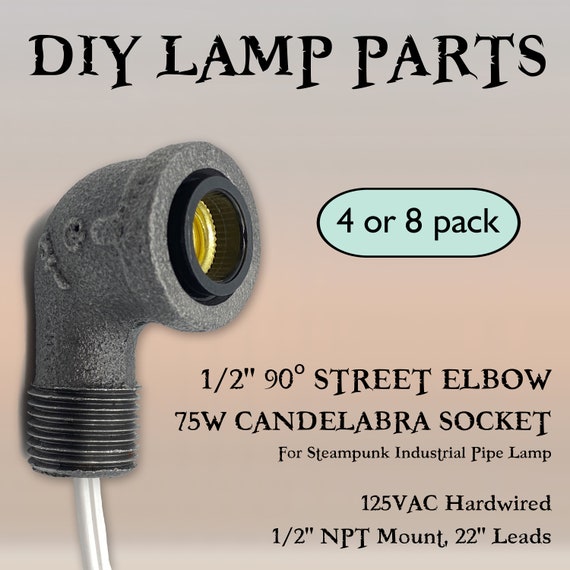This image features an infographic titled "DIY Lamp Parts." At the top of the image, the text "DIY Lamp Parts" is prominently displayed in black. Beneath this, there is an image of a gray elbow-shaped socket, resembling an L-joint pipe with a screw base on one end and a white wire protruding from the other end. Adjacent to this socket is a blue oval text box outlined in black, containing the text "4 or 8 pack." Below this, there is detailed information about the parts, reading: "1.5 inch 90-degree street elbow, 75W candelabra socket for Steampunk Industrial Pipe Lamp, 125VAC hardwired, 1.5 inch NPT mount, 22 inch leads." The background consists of three pastel-colored layers, with the top layer in a muted hue that vaguely resembles purple, and the middle layer an orange shade, contributing to the visual appeal and structure of the infographic.